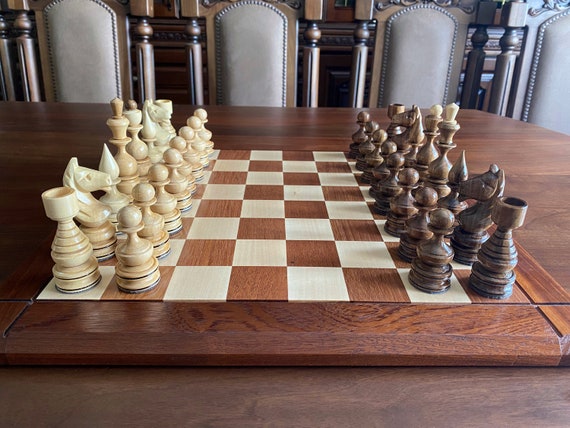This photograph captures a meticulously arranged wooden chess set viewed from the side. On the left side of the board are the white pieces, while on the right are the black pieces, each perfectly aligned in their starting positions. The board and the pieces are crafted from wood, exuding a classic and elegant feel. The setup rests on a polished, dark wood table, enhancing the set's traditional aesthetic.

In the background, three intricately carved wooden chairs with ornate designs frame the scene. These chairs feature green cushioning on their backs, adding a touch of color and elegance to the setting. The chess pieces, though conventional, have unique characteristics: the knights are distinctly knight-like, the rooks resemble traditional castles, and the bishops feature teardrop-shaped tops. Overall, the image exudes a sense of timeless strategy and old-world charm.